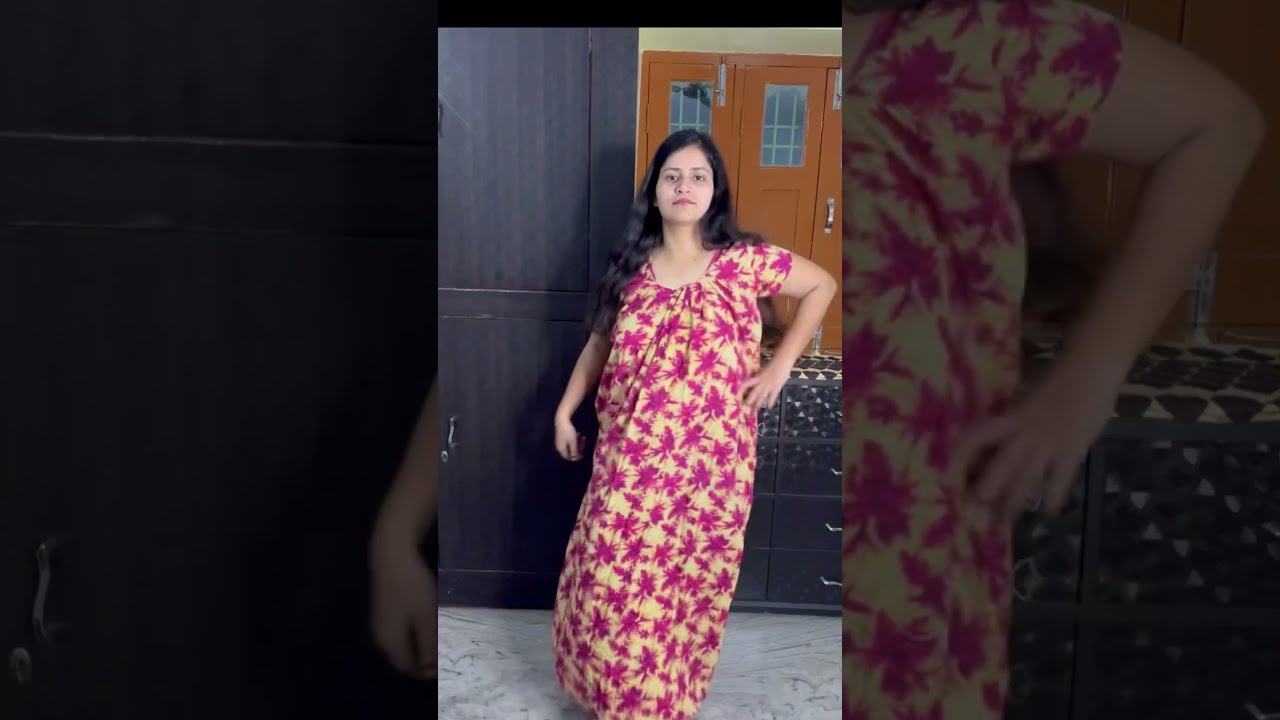In this split-screen image, a woman, potentially of Indian descent, stands poised in the center of a living room, her feet slightly cut off from the frame. She wears a long, tan-colored dress adorned with bright pink and red palm tree patterns and hints of yellow and orange. The woman has long, dark hair and gazes directly at the camera with a neutral expression. Her left arm is bent, hand resting on her hip, while her right arm dangles naturally by her side. Behind her, a closed brown door and dark brown cabinets are visible, potentially reflected in a nearby mirror. The floor beneath her is gray carpet. Elements of the room, such as black furniture, contribute to the overall color palette consisting of tan, pink, black, gray, white, orange, brown, yellow, and hints of blue.